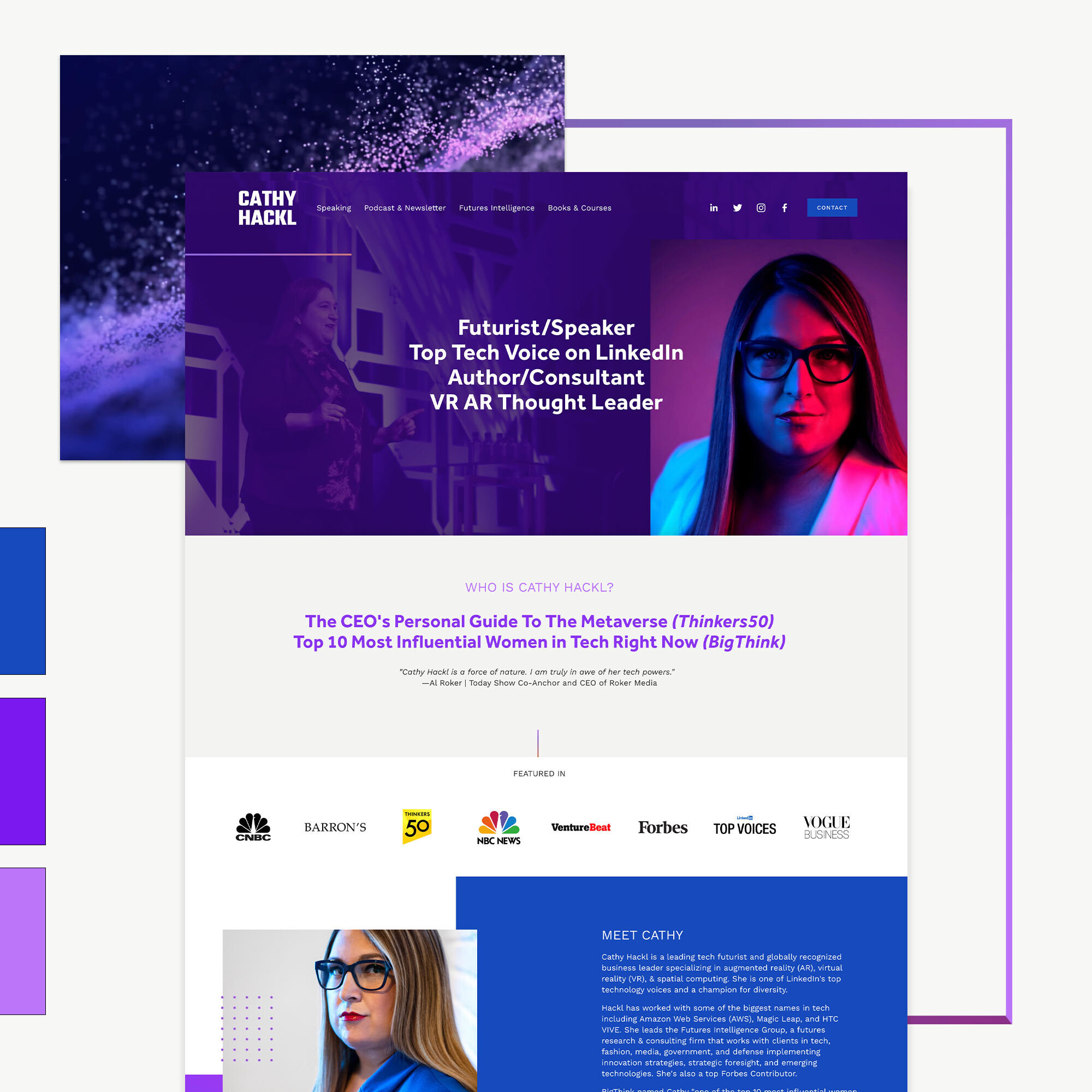The image features a layered pop-up collage, primarily set against a gray background with vertical and horizontal purple lines accentuating the right side. At the top, a predominantly purple pop-up showcases a slightly eerie-looking woman on the right side. She has brown hair and black glasses. 

The left part of this pop-up is white, displaying text that reads: "Kathy Hepburn. Speaking Podcast, Newsletter, Feature, Intelligent Book and Courses. Futurist/Speaker, Top Tech Voice on LinkedIn, Author/Consultant, VR/AR Thought Leader." 

Beneath this, a gray and purple striped background carries text stating, "Who’s Kathy Hepburn? The CEO's personal guide to the metaverse and a top thinker on Thinkers 50's list of the 10 most influential women in tech right now. A big thank you." Followed by a black text quote: “Kathy Hepburn is a force of nature. I am truly in awe of her tech powers.” - Al Roker, Today’s Show Co-Anchor, CEO of Roker Media.

Below, logos of prominent companies where she has been featured are displayed, including CNN, Barron's, NBC News, VentureBeat, Forbes, Top Voices, and World Business.  

At the bottom, against a dark bluish-black background, the text reads: "Meet Kathy." In the upper left-hand corner of the entire collage, a rectangle containing different shades of blue and purple is placed, enhancing the visual diversity.